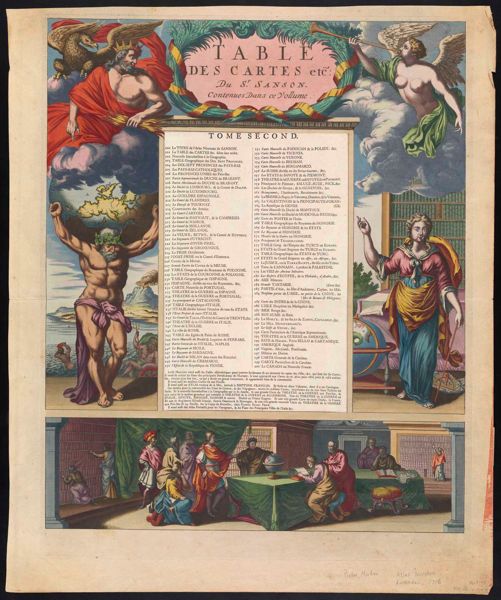The image is a photograph of an old, framed poster, likely from a middle-aged or Renaissance-style publication. It features colorful artwork depicting various mythological and religious figures. Dominating the center of the poster is a large volume of text on a white paper, titled "Table de Cartes, etc.," enclosed in a pink oval that reads "Tome Second." Above this central text, on the left, stands a crowned man holding a harpy, while on the right, an angel with white wings and a trumpet. Below the title, a nearly naked figure of Atlas strains under the weight of the planet on the left side, and a woman in a red and blue dress points at a list of items on the right. At the bottom of the image, a detailed scene shows various individuals seated around a table, examining books, a globe, and maps. The whole poster is enriched by a palette of black, tan, red, green, yellow, blue, and white, suggesting the work's age and intricate detail. The overall setting appears to be reminiscent of an old magazine or newspaper page.